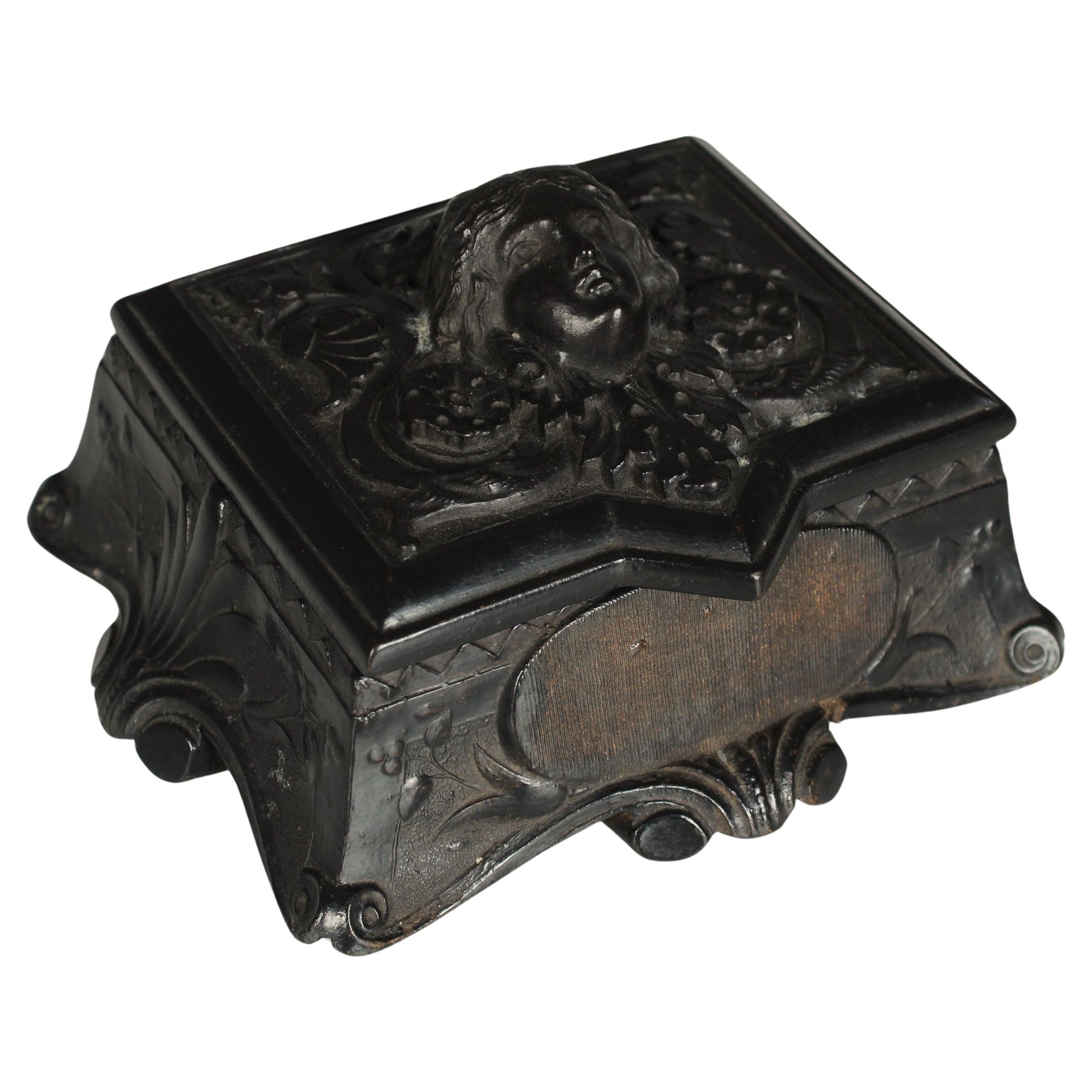This close-up image showcases a beautifully crafted decorative box that appears to be made of metal, possibly brass or bronze, antiqued to a dark, almost black finish with hints of brown where the paint has worn thin. The box features an intricate design with baroque elements. The top of the box prominently displays an extrusion of a woman's head with neck-length hair, seemingly laying her head against the box lid, face down. An intricate pattern surrounds the woman’s head, adding to the ornate aesthetic.

Both the front and sides of the box are adorned with detailed floral embroidery, with the front also featuring a small, widened brown circle at its center. There is a triangle pattern running along the top edge, formed by alternating up and down triangles, visible all the way around. The corners of the box are rounded and tapered, giving it a sculpted appearance with pointed outward edges, while the front and sides are gently tapered inward, preventing a squared-off look.

Overall, the box exudes a vintage charm, reminiscent of a carved wooden jewelry or cigar box, characterized by its combination of intricate design, metalwork, and carefully executed patterns.